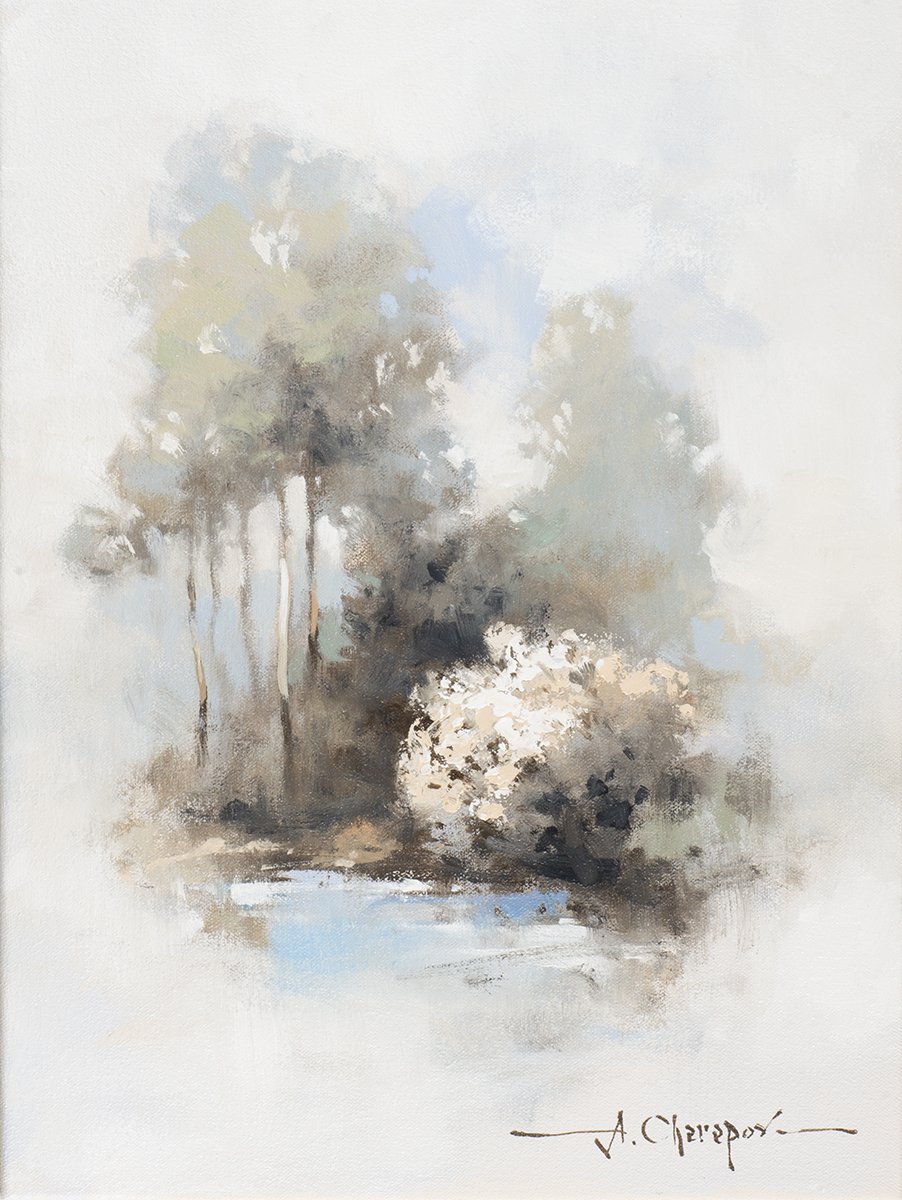This image is a painting that showcases a serene forest clearing dominated by tones of white, very light blue, grey, and brown, suggesting a calm and peaceful atmosphere. The central focus of the painting includes a cluster of slender trees with whitish-brown trunks and a sparse arrangement of green leaves, suggesting a mix of trees in varying seasonal stages. To the right and in front of these trees, there are bushes painted in shades of brown, black, and green, and an orange bush, creating a layered natural scene.

In front of the bushes lies a small, light blue patch of water, possibly a pond or lake, adding a reflective element to the composition. The background and much of the canvas is predominantly white, with hints of blue that might represent the sky peeking through the foliage. The sky is depicted with subtle white clouds and spaces of blue in between, blending softly into the scene.

The composition appears as a combination of delicate brush strokes or smudges, suggesting it might be created with watercolors or oils, lending it a fluid, almost impressionistic quality. The painting occupies about two-thirds of the central canvas, with the edges remaining mostly white, enhancing its minimalist feel.

The bottom right corner of the painting features the artist's signature, signed in dark brown ink. The signature reads "A. Cherrapas," though there is some uncertainty about the exact spelling. Overall, the tranquil and subdued tones of the painting, combined with its soft execution, evoke a quiet, reflective mood.